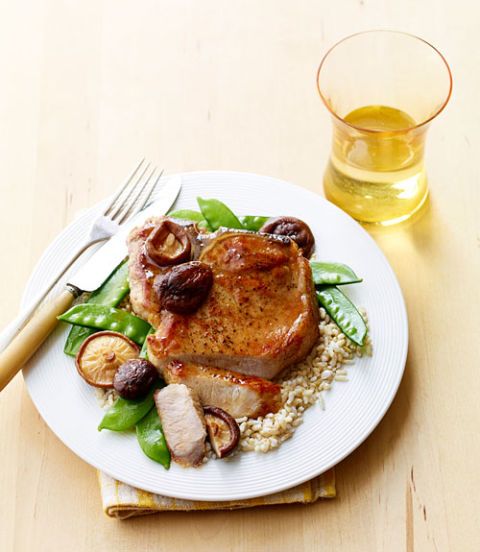The image showcases a detailed close-up of a gourmet meal presented on a white plate that almost spans from the left middle to the bottom of the frame. The centerpiece of the dish is a golden-glazed pork chop, from which two slices have been neatly cut and placed nearby. The pork chop is artfully arranged over a bed of coarser grains, possibly quinoa or pilaf, which has a subtle white-green hue. Accompanying the pork chop are five shiitake mushrooms and a handful of fresh, green snap peas. The mushrooms are strategically placed around the plate, while the snap peas form a semicircular arrangement to the left and right.

The table setting includes a fork and a wooden-handled knife positioned on the right side of the plate, with the knife closest to the food. The plate itself sits atop a yellow and white striped napkin, indicating a casual yet thoughtfully arranged meal scene. To the upper right of the image, a unique glass with an amber hue and a pinched middle holds a light yellow liquid and is about a third full.

The meal and glass are set on a natural wood table, which provides a rustic backdrop. Softly faded colors in the background contribute to a serene and inviting dining atmosphere.